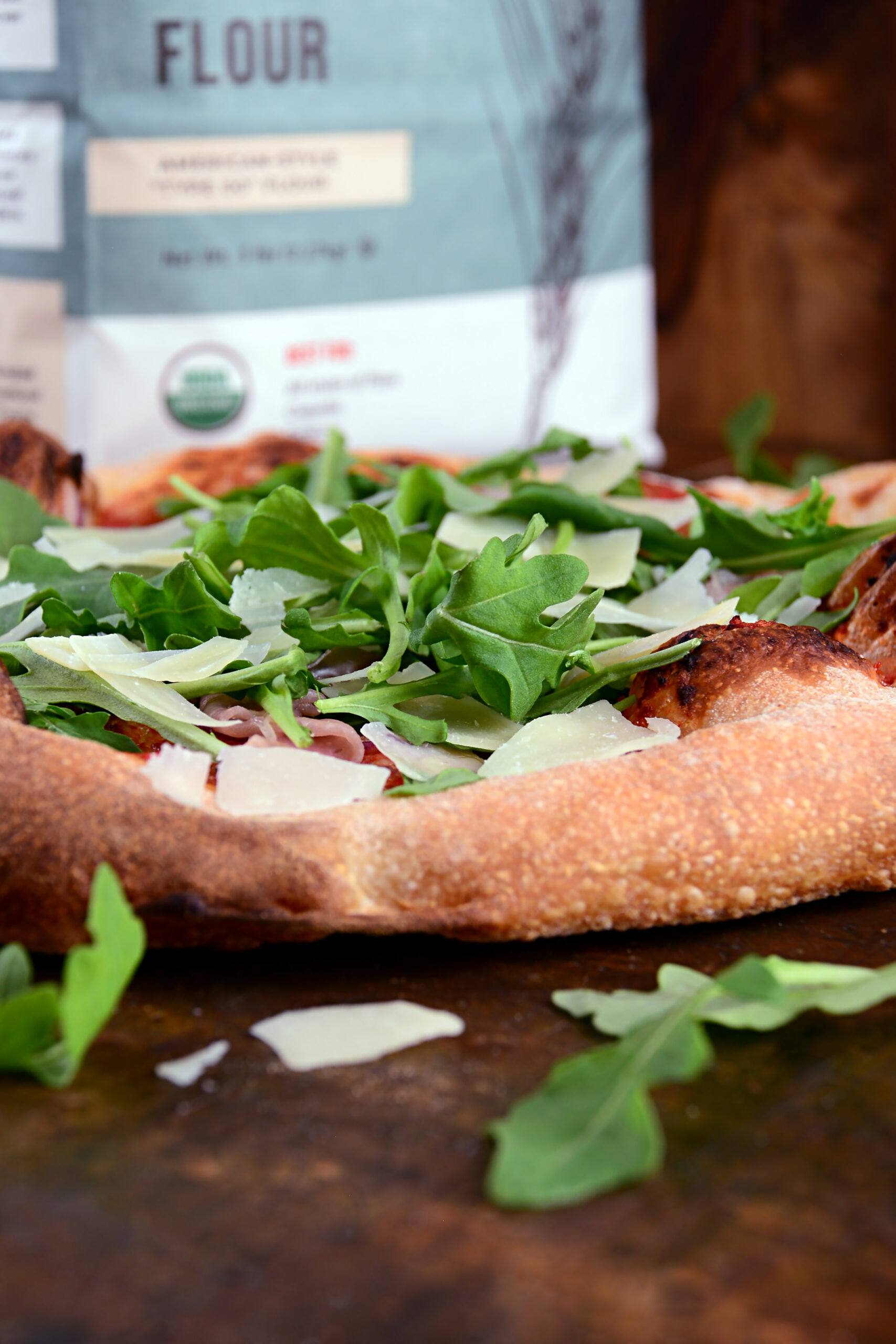In this detailed image, we see a freshly cooked pizza with a slightly burnt, brown crust, beautifully presented on a dark wood table. The pizza features vibrant green arugula and spinach leaves with visible stems, as well as generous shavings of Parmesan cheese delicately laid on top. Red tomato sauce peeks through, complementing the slices of folded ham or prosciutto that add a savory touch. Scattered within are thin rings of onion, further enhancing the pizza’s flavor profile. Beside the pizza, the same ingredients, including Parmesan shavings and green leaves, can be seen on the table. In the background, a blue and white bag of flour marked "flower" adds a rustic touch to the scene.